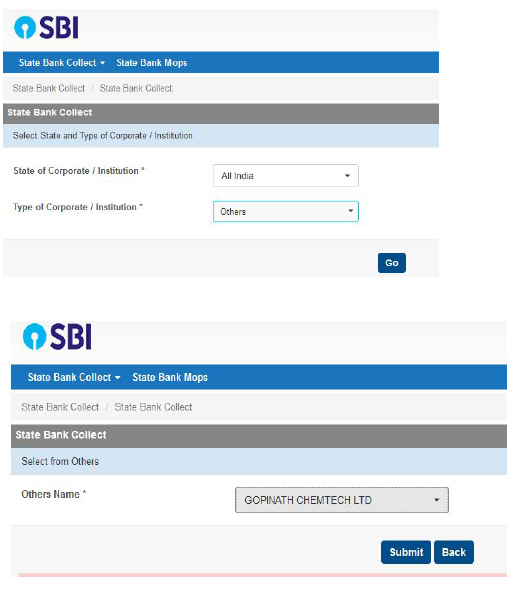The image comprises two separate screenshots from a banking platform website, presumably associated with the State Bank of India (SBI). 

In the first screenshot, at the very top, there is the SBI banking logo, identifiable by its acronym. Directly beneath the logo, a prominent blue navigation bar displays an option labelled "State Bank Collect" with an adjacent drop-down menu, alongside a sub-menu labeled "State Bank Maps." Below this blue bar is a grey toolbar designed for user interaction, featuring a selection for "State Bank Collect." This section includes drop-down boxes for users to select the "State" and "Type of Corporate/Institution." In this instance, "All of India" is selected in the state dropdown box, while "Others" is chosen in the type of corporate/institution dropdown. A "Go" button is situated nearby to advance to the next page.

The second screenshot depicts the subsequent page following the interaction. This page largely mirrors the previous one but introduces a new dropdown selection titled "Select from Others." Here, the option "Gopinath Chemtech LTD" is chosen, likely narrowing down the corporate/institution field based on the user's prior selections.

Both screenshots offer a step-by-step walkthrough of navigating the SBI banking platform to facilitate specific corporate or institutional transactions.